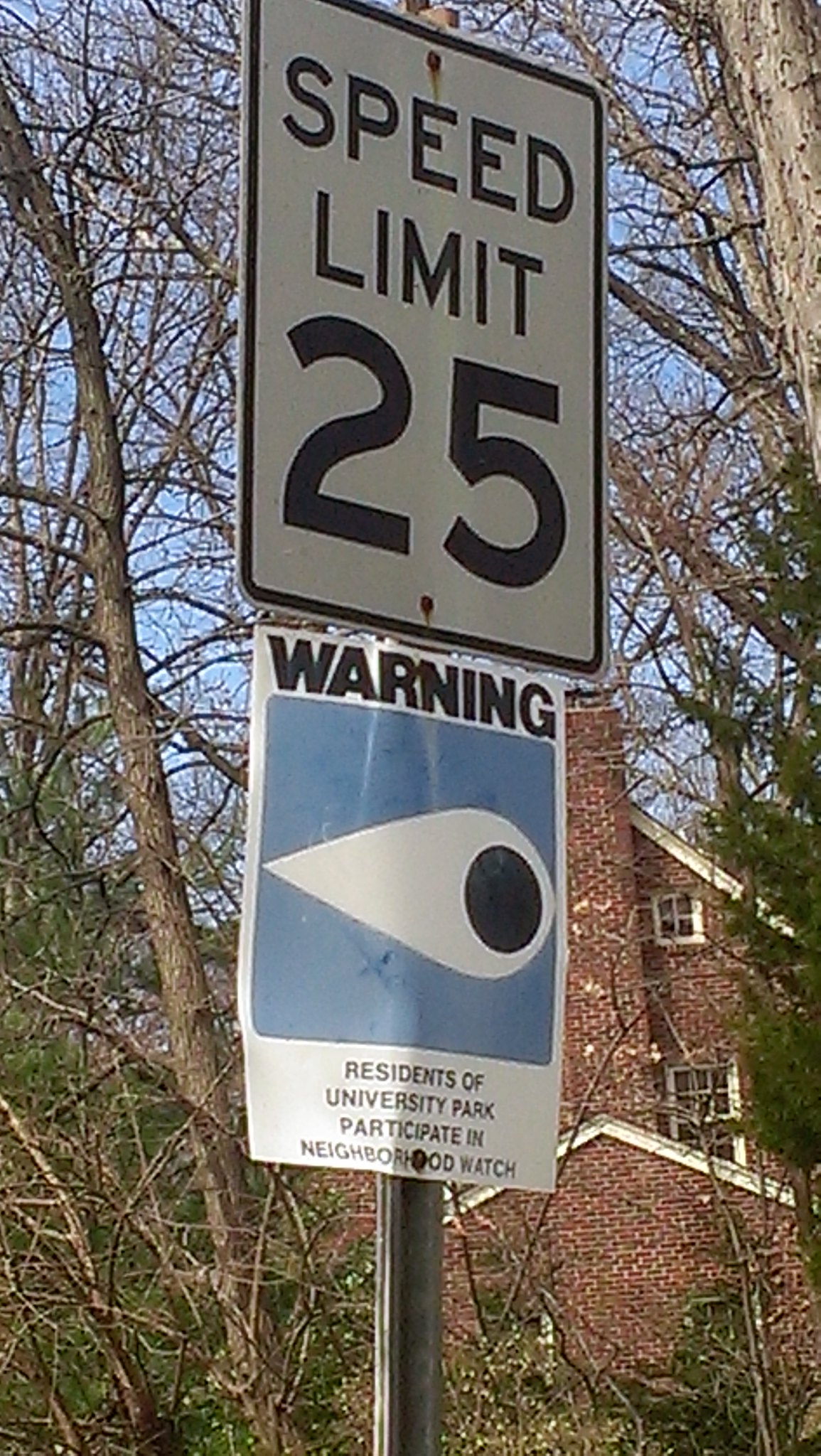This photograph, taken on a sunny day, features a metal pole with two signs attached to it, standing prominently in the foreground. The top sign is a weathered, rectangular white traffic sign with a black border, displaying "Speed Limit 25" in black letters. Rust stains are visible, indicating it has been in place for a considerable time. Below, there is a flimsier white sign featuring a blue square with a white, teardrop-shaped eye that has a red dot in the center. The black text on this sign reads, "Warning, residents of University Park participate in Neighborhood Watch."

In the background, a large, red brick three-story house with a tall chimney and white-framed windows is visible. The edge of the roofing is highlighted in white, contrasting against the red brick. The house appears to have either a garage or an extension on one side. Surrounding the house, most of the picture is filled with the empty branches of deciduous trees, suggesting that it is likely winter. Additionally, there is a pine tree encroaching from the right-hand side of the image and some shrubs at the bottom, adding to the wintry scene.